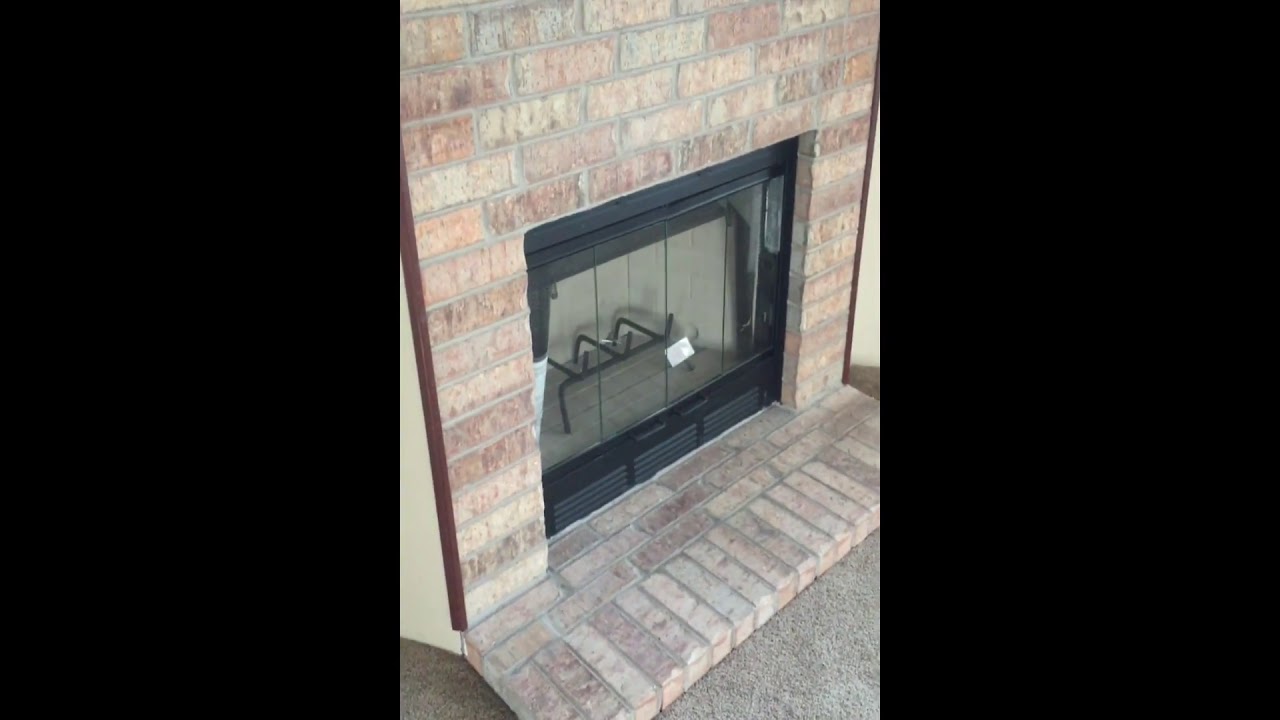The photograph captures an old, narrow, and tall indoor fireplace bordered by long vertical black bars on both sides. The fireplace is constructed from red bricks dulled with age, with gray mortar in between. The surrounding walls are beige and the floor is a grayish-brown hue. The fireplace itself is fronted by a see-through glass grate with two small handles and ventilation slots beneath it, suggesting it is an electric fireplace designed to hold logs on a wrought iron rack inside. Inside, the fireplace features bricks in a tan color, with a piece of paper or a white sticker attached, indicating it may be new. The fireplace cover has a distinct black border. Overall, the image is in color, clear, and appears to be taken during the daytime with ample natural lighting. There are no people, animals, words, or numbers visible in the image.